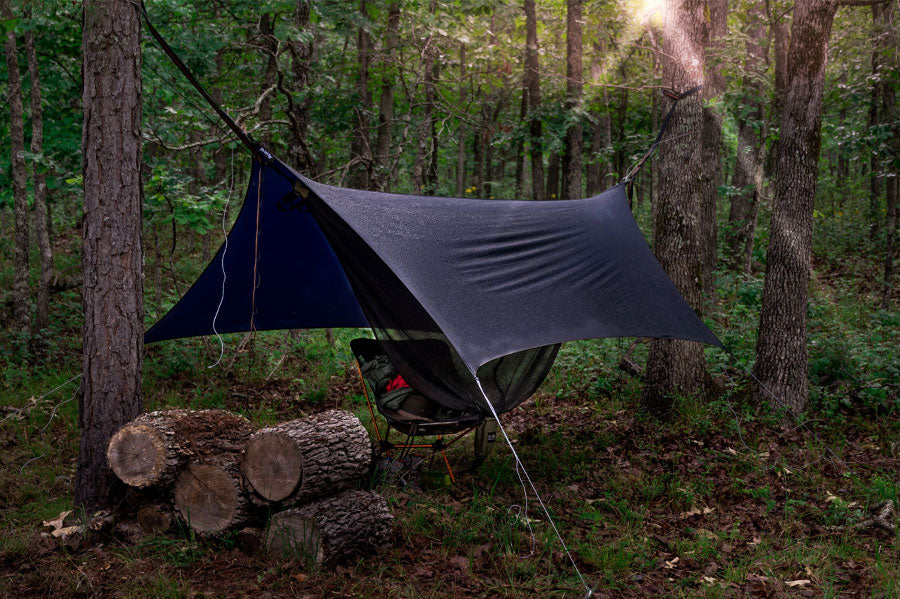This detailed close-up image captures a serene forest campsite. Suspended tautly between two slender trees is a blue tarp, anchored securely to the ground at each corner with small white strings. Beneath the tarp, a black folding chair is positioned, hinting at a cozy setup for relaxation. Stacked neatly at the base of one of the trees are four thick wooden logs, precisely chopped and ready for use. The forest floor is a natural tapestry of grass and leaves, with scattered wood shavings and dirt adding to the rustic feel. In the background, the dense forest stretches out with numerous trees, and bright sunlight filters through, with radiant sunbeams creating a dappled effect in the upper right corner of the picture.